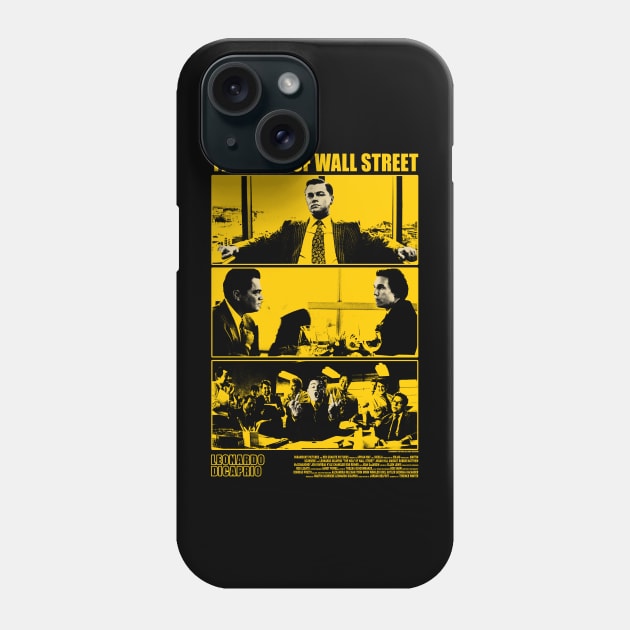The photograph depicts the back of a black smartphone with curved edges, showcasing a rectangular shape. In the upper left corner of the phone, within a small square, there are two camera lenses and a flash. One lens is positioned in the top left corner of the square, and the other in the bottom right. Opposite to each lens, there are small circles; a white one in the opposite corner of the top left lens, and an even smaller black circle opposite the bottom right lens.

Mounted on the back of the phone is a black and yellow poster for the movie "The Wolf of Wall Street." At the top of the poster, in yellow lettering, are the words "Wall Street," though the preceding text is obscured. Below this text is an image of Leonardo DiCaprio, presumably from the film. Underneath DiCaprio's image, there are two additional scenes from the movie: one of two actors seated across from each other, and another featuring several people with one individual in the center, mouth open, facing the viewer.

At the bottom left of the poster, the name "Leonardo DiCaprio" is printed in yellow, with more tiny yellow text on the lower right corner, though it is too small to be legible.